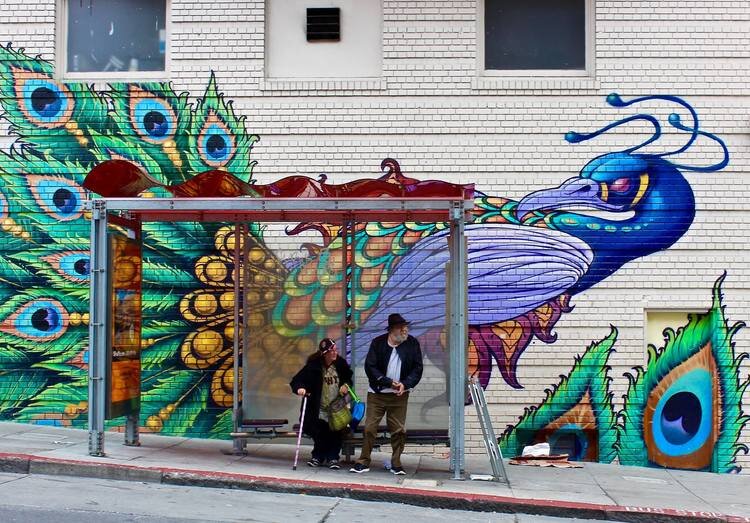In this outdoor photograph, the scene captures a concrete sidewalk bordered by a road at the bottom. Centrally placed on the sidewalk is a bus stop, featuring two individuals awaiting their bus. On the left, a woman is seated, clad in a black jacket, black pants, and black-and-white sneakers, topped with a black and white cap. On the right, a man stands, dressed in a dark sweater, brown pants, and dark shoes. Both individuals gaze rightward.

Behind the bus stop, a large white wall of a building serves as a backdrop, adorned with a vibrant piece of street art. The mural showcases a multi-colored peacock, with its head painted blue, wings in purple and green hues, and a tail in striking shades of yellow, lime green, and blue. The wall also features a couple of windows, enhancing the urban essence of the setting.